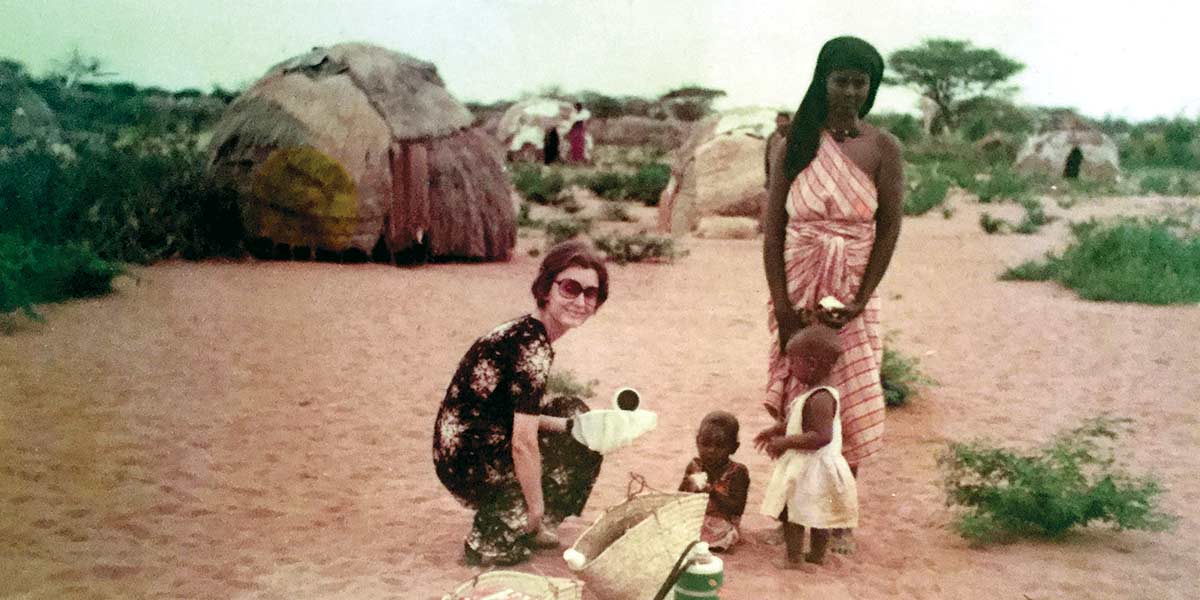In this evocative photograph, taken outside an indigenous African village, a harmonious blend of cultures is prominently featured. The ground, a rich terracotta dirt with patches of sporadic green ground cover, sets the natural backdrop. At the center of the scene, a Western woman with ear-length brown hair crouches down, her floral dress fluttering slightly. She wears dark sunglasses and gazes directly at the camera, her posture open and engaging.

Next to her, two young African children capture the essence of innocence and tradition. One girl, dressed in a pristine white dress, stands poised while another girl, adorned in a vibrant flower-patterned dress, sits calmly on the earthy ground. Beside her rests a large straw basket and a green canteen, suggesting a scene of daily life and utility.

Standing protectively behind the girl in the white dress is their mother. She exudes grace and strength in a one-shouldered dress fashioned from a red and white striped wrap, a testament to the intricate textile traditions of her culture. The backdrop reveals a cluster of huts constructed from intricately layered mats in various shades of tan, gray, and reddish hues, reflecting the diverse and resourceful materials provided by their environment.

This image captures not just a moment in time but a vibrant tapestry of cultural intersections, familial bonds, and the enduring spirit of the village.